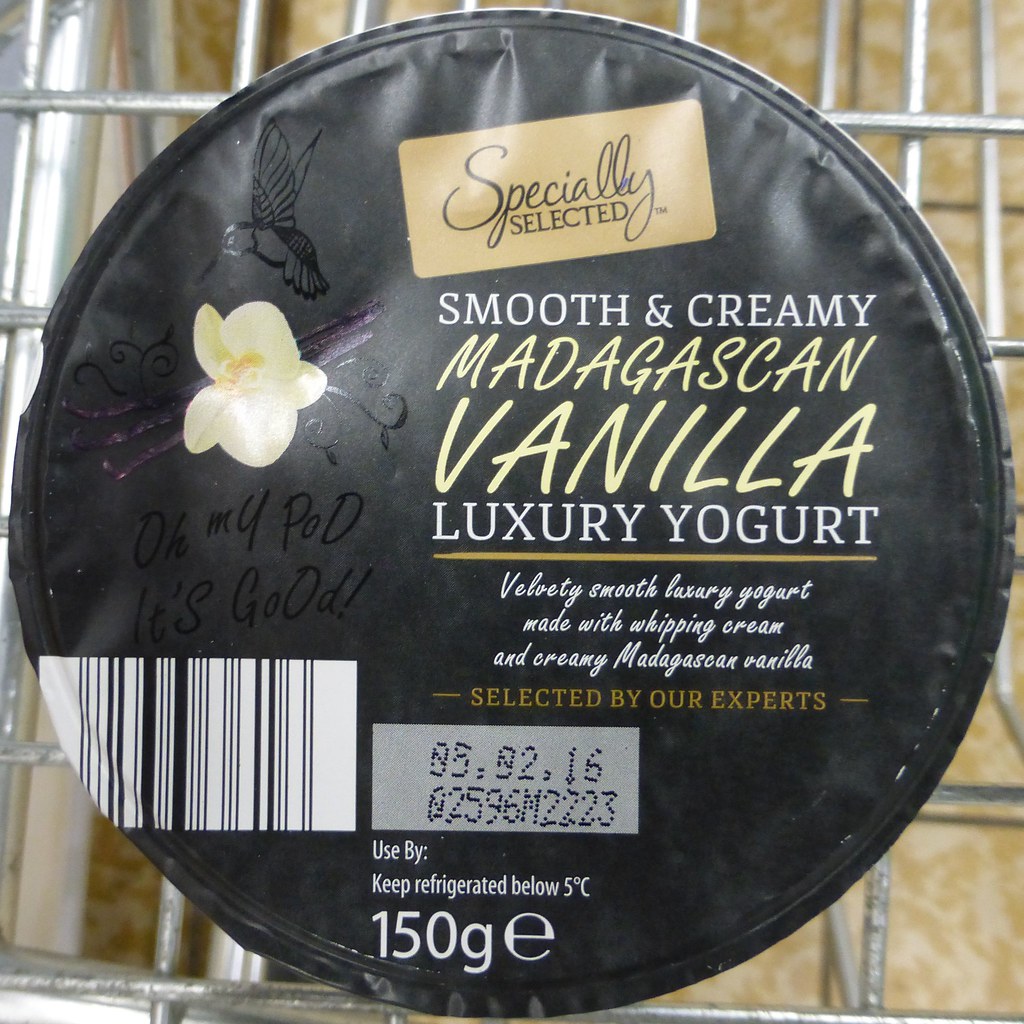The image is a top-down photograph capturing a small circular pot of yogurt, positioned on a shopping cart with a beige countertop faintly visible through the metal grates. The yogurt container features a black lid prominently labelled with a gold badge that reads "Specially Selected." The text on the lid is a mix of white and yellow, stating "Smooth and Creamy Madagascan Vanilla Luxury Yogurt." Additional details on the label emphasize its premium nature, mentioning "Velvety smooth luxury yogurt made with whipping cream and creamy Madagascan vanilla, selected by our experts." On the left side of the lid, there is an illustration of vanilla bean stalks and a small flower. The barcode is also visible, along with a whimsical phrase "oh my pot, it's good." The yogurt weighs 150 grams and must be kept refrigerated below 5 degrees Celsius. The photo captures the luxurious branding and textures of the container against the utilitarian backdrop of the shopping cart.